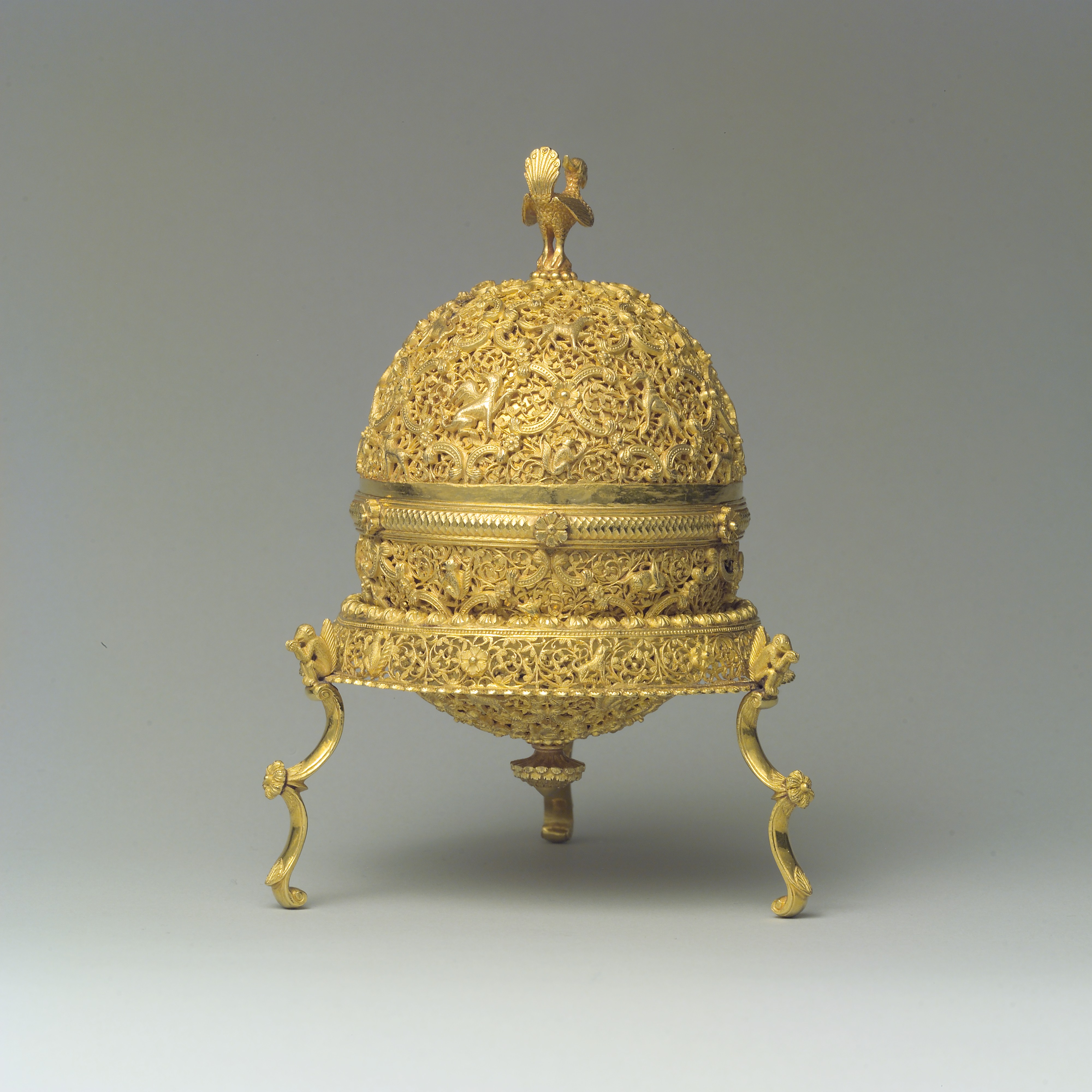The image depicts an opulent golden egg, evocative of Aladdin, Persian and Turkish royalty, and Indiana Jones. This magnificent container is set against a grayish, creamy backdrop. It possesses three exquisitely filigreed legs, which appear to be adorned with intricate angelic figures and delicate ribbons. The egg, almost perfectly rounded rather than oblong, features a central gold band reminiscent of a zipper, embellished with tiny carved flowers in a zigzag pattern, with three prominently visible on the sides and front. Nestled within another intricately filigreed frame, the egg's base and the top are opulently designed, with the top boasting a bird-like golden handle. This handle showcases the bird's tail flipping upwards, with two elegantly curved wings bending downwards on either side. The entire piece casts a shadow on the contrasting white and gray background, enhancing its elaborate and expensive appearance, making it not just a container, but a luxurious decorative artifact.